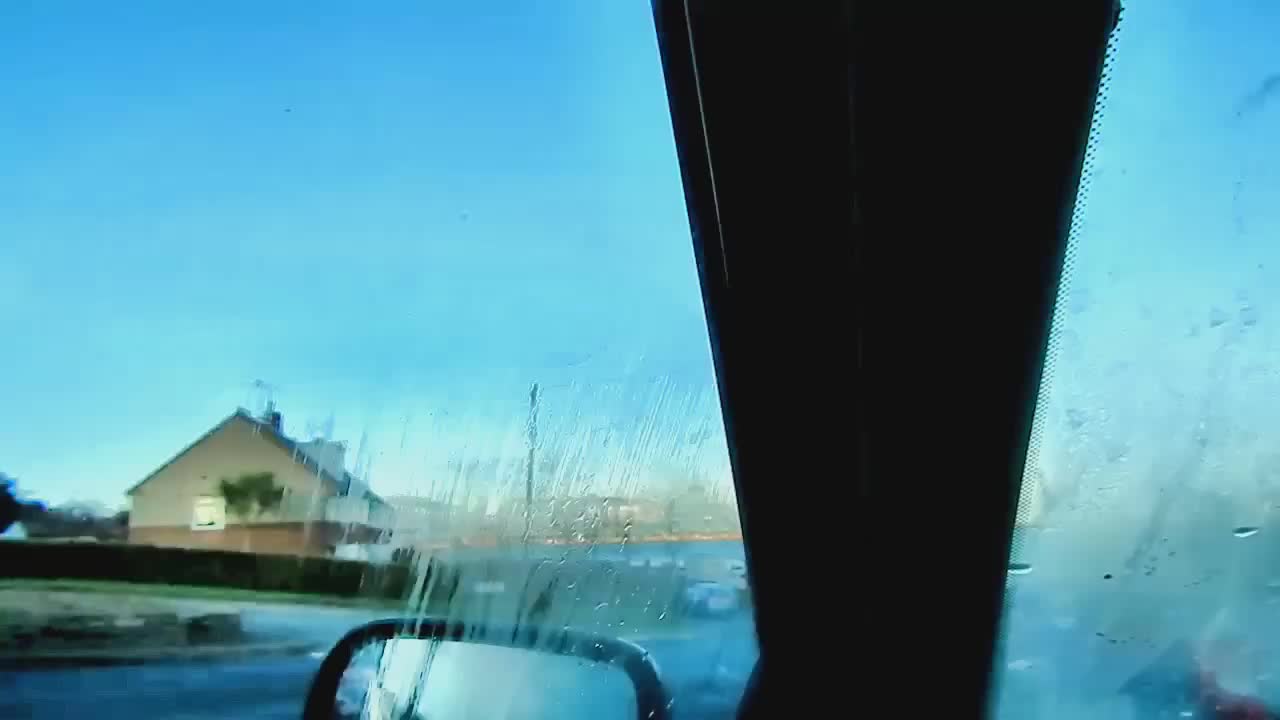A low-quality, out-of-focus photograph taken from within the driver's seat of a vehicle captures a peculiar perspective. The focal point of the image is the black metal pillar, or A-pillar, situated between the windshield and the driver's side window. On the lower left, slightly off-center, part of the driver's side mirror is visible, framed by black metal and featuring a rounded-rectangular shape with smooth edges. To the right, a narrow section of the windshield can be seen, entirely obscured by a layer of frost and ice.